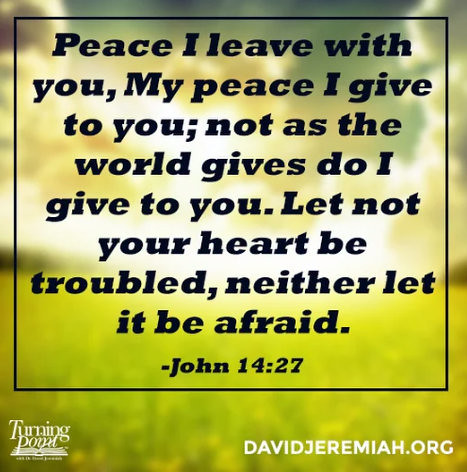The image appears to be a frame from a PowerPoint presentation featuring an out-of-focus background image of a grassy meadow under a cloudy sky. At the center, there is a black-bordered box containing a prominent Bible verse in large, bold, black print: "Peace I leave with you, my peace I give to you, not as the world gives do I give to you. Let not your heart be troubled, neither let it be afraid. - John 14:27". In the lower left corner, there is a logo for Turning Point Ministries that incorporates a stylized Bible. In the lower right corner, there is the URL davidjeremiah.org. The overall color scheme includes green and white from the background, contrasted by the bold black text.